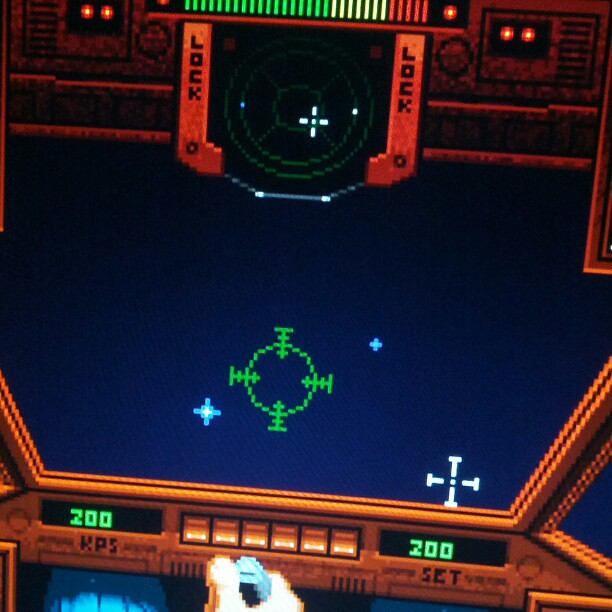This screenshot captures a vintage pixelated video game that appears to be set inside a spacecraft cockpit. The scene features a hand, with a white skin tone, operating a light blue joystick at the bottom of the image, possibly controlling the ship. The interior of the spaceship is visible, showcasing intricate details such as the left and right walls, windows, and key instrumentation. 

Prominently displayed in the middle is a circular green crosshair with four points extending outward (left, right, up, and down), indicating targeting capabilities. The background is a depiction of space, adorned with blue star-like objects scattered across the top left and right, and bottom left and right quadrants.

Textual elements include green numbers '200' displayed on both the bottom left and right inside black rectangles, with 'KPS' underneath the left and 'S.E.T.' underneath the right. Above, at the top, are two red vertical tabs, each labeled 'LOCK'. Also present is a graphical bar indicator system, with most bars showing green, some yellow, and few red, likely depicting the health or energy status of the ship.

The overall ambiance and graphical style are reminiscent of classic arcade space shooter games, where pixelated visuals and straightforward interface elements dominate the screen.